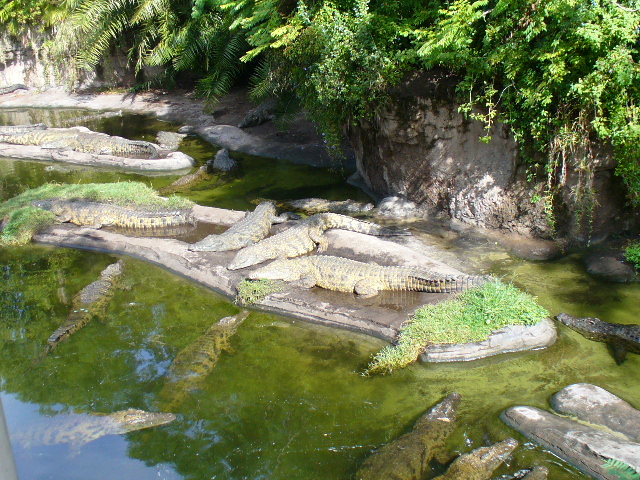This outdoor image captures a bustling crocodile habitat, possibly within a zoo or dedicated sanctuary. Central to the composition is a large body of murky, greenish freshwater, surrounded by rocky formations and lush green foliage. The water reflects a clear blue sky, enhancing the scene's natural beauty. Numerous crocodiles, at least a dozen, can be seen lounging on flat, sunlit rocks and in the water. Their light gray bodies, tinged with green and black, blend seamlessly with the surrounding environment. The crocodiles are scattered throughout the habitat: some are sunbathing on a central rock island covered with grass and moss, while others navigate through the water or rest near boulders at the bottom right of the image. The rocky shoreline and a backdrop featuring a rock wall adorned with vegetation frame this dynamic and serene landscape.